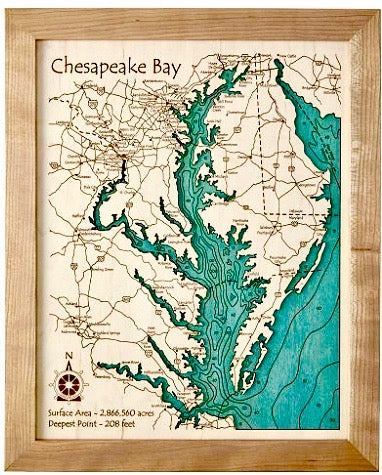The image features a topological map of the Chesapeake Bay encased in a wooden picture frame. The mainly white map is intricately detailed with black lines representing roads and a turquoise-colored depiction of the Bay’s waters. In the top left corner, brown text spells out "Chesapeake Bay." A compass, designed to resemble an old-fashioned wooden captain’s wheel, is positioned in the bottom left corner with the letter "N" denoting North. Beneath the compass, black lettering states the Bay's surface area as 2,866,560 acres and its deepest point as 208 feet. The map's beige brown backing adds a subtle contrast to the overall design.